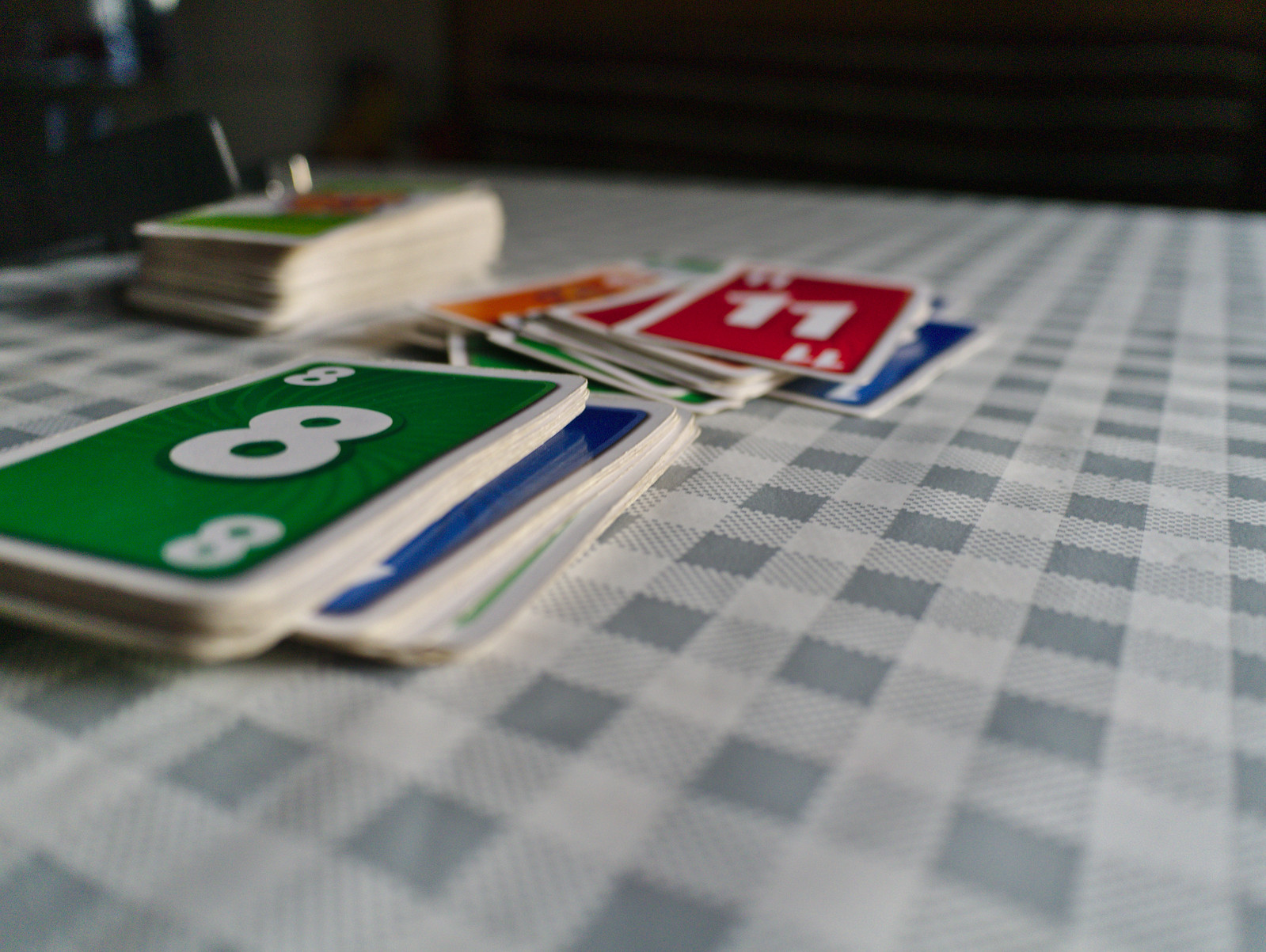In the image, a table with a detailed checkerboard pattern occupies the majority of the frame. The tablecloth features an intricate design, consisting of gray, white, and light gray squares. White vertical lines cross the tablecloth, intersecting with blue horizontal lines, creating a striking checkerboard effect.

Scattered across the table are several Uno cards. In the center-left of the image, a prominent green Uno card with the number 8 is visible, showcasing a large '8' in the center and smaller '8's in the upper left and lower right corners, though the lower right '8' appears slightly blurred. Partially hidden beneath this card, a blue Uno card peeks out. Nearby, a red Uno card marked with the number 11 is identifiable, though the '11' in the upper left corner is blurred.

The cards are not neatly arranged, revealing glimpses of additional red, blue, green, and orange Uno cards, hinting at a recently halted game. A chair is positioned in the distant corner of the frame, suggesting a casual, perhaps paused moment in an otherwise engaging card game.

The overall composition is tightly focused on the table, leaving little visible of the surroundings, thus drawing the viewer’s attention to the vibrant combination of colors and patterns presented on the table.